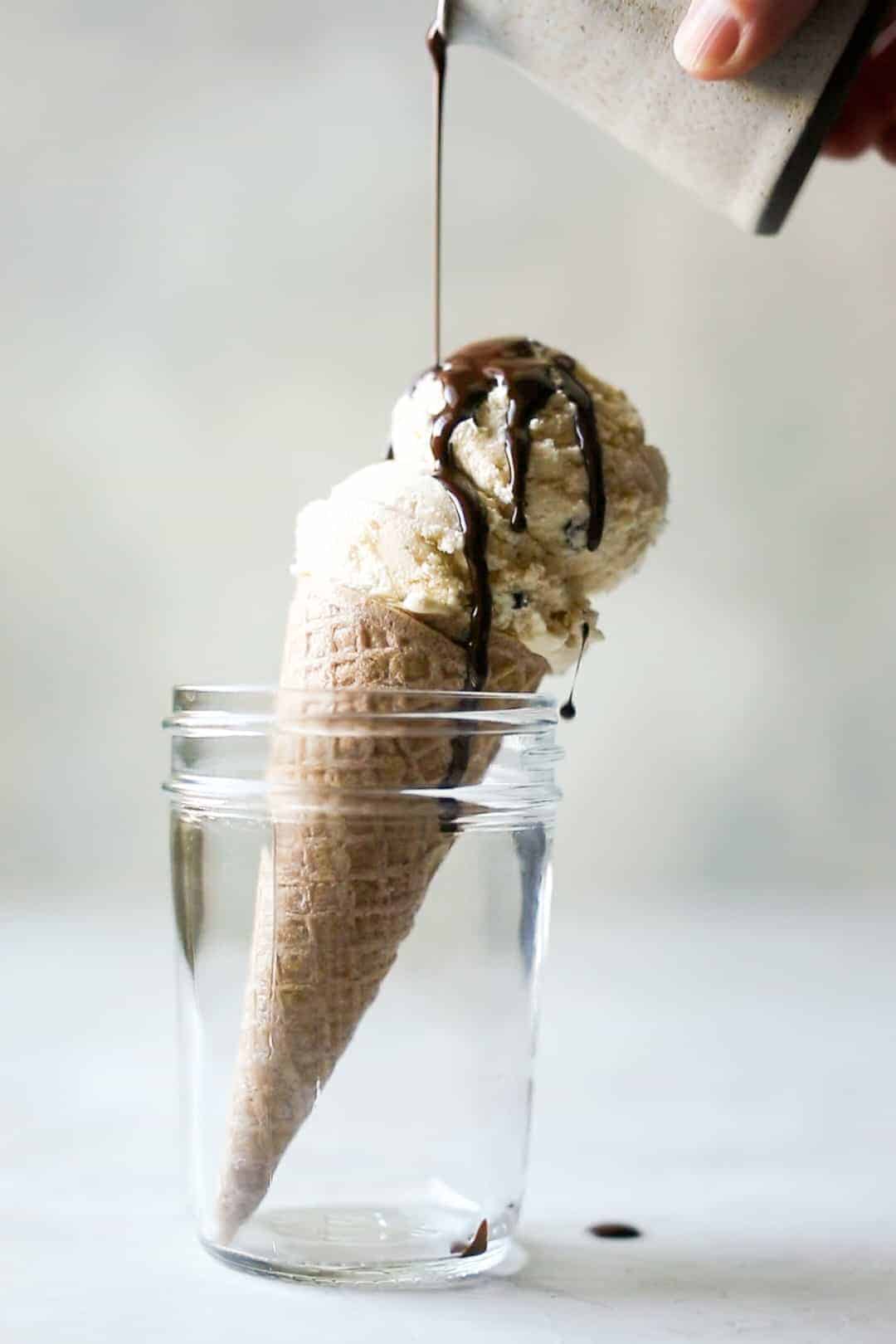In this detailed studio shot, the focus is on an ice cream cone nestled in a transparent short pint mason jar. The jar is central to the image, with the cone leaning to the right. Two scoops of vanilla ice cream, speckled with tiny chocolate chunks, fill the waffle cone. From just outside the top right of the frame, a hand appears, pouring rich, glossy chocolate syrup from a ceramic cup or packet. The syrup cascades down the ice cream, creating a delightful drizzle. A small spot of this chocolate syrup has puddled on the blurry white surface beneath. The entire scene is set against an off-white, slightly gray, and softly lit background, typical of studio photography, enhancing the visual appeal of the deliciously detailed treat.